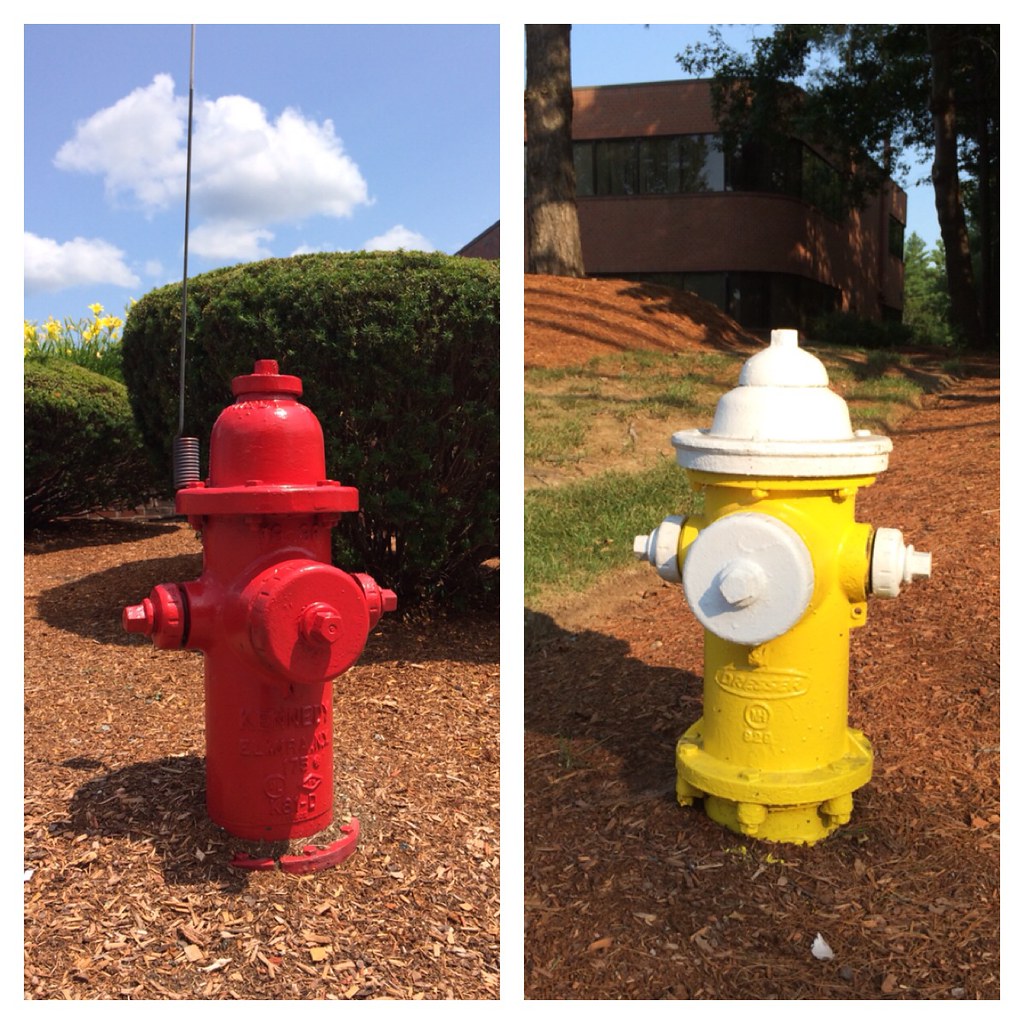The image is divided into two side-by-side, rectangular, portrait-shaped photographs, both showcasing fire hydrants on a brown mulch floor. The left photo features a bright red fire hydrant with an antenna-like gray rod extending upward into a blue sky filled with some clouds. Surrounding the hydrant are a large, well-trimmed hedge with yellow flowers peeking over, and two bushes. The right photo shows a yellow fire hydrant with a white top and round white protrusions in the middle. The background includes a slightly green hill, trees on both the left and the right, and portions of a brick building with large rectangular windows facing the camera. The sky in this photo is also blue, complementing the overall scene.